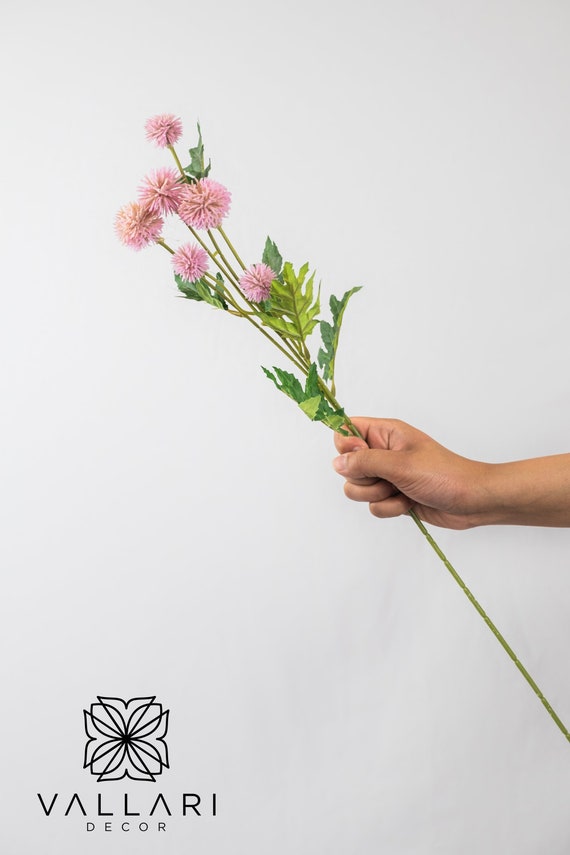The photograph showcases a human hand extending from the right side of the frame, holding a slender green stem. This stem, adorned with a few leaves resembling maple or oak leaves, ascends to reveal six small, spherical, pink flowers, each about the size of a dandelion. The background is a very light gray, almost white. In the bottom left corner, the text "Vallaria Decor" is presented, with "V-A-L-L-A-R-I-A" clearly spelled out. Above this inscription is a stylized black symbol reminiscent of four intersecting pyramids forming a clover-like design.